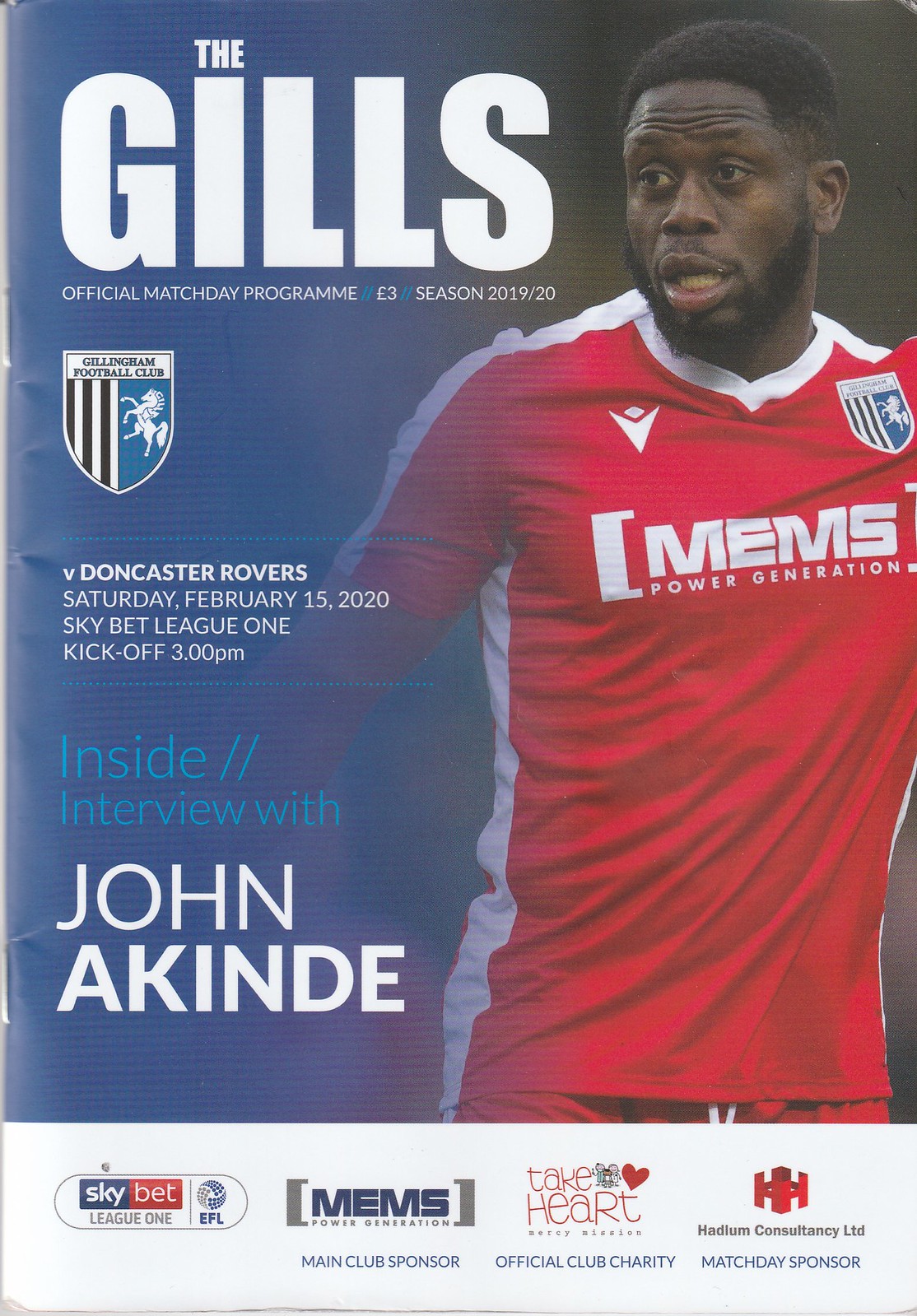The cover of the Gills Official Match Day Program for the 2019-2020 season prominently features a bold title "THE GILLS" at the top. Below, in white text, it states "Official Match Day Programme" priced at three pounds. The background is split into a blue left half and a black right half. A central image showcases an African American male soccer player, presumably John Akinde, donning a red jersey with white detailing and the text “MEMS Power Generation.” On the left side, details about an upcoming match are noted in white: "Vs Doncaster Rovers, Saturday, February 15th, 2020, Sky Bet League One, Kickoff 3 p.m." Additionally, the cover highlights an interview with John Akinde specified in a mix of white and blue text. The program also includes a shield logo with a horse in blue, white, and black stripes, representing the team’s emblem. At the bottom, various logos denote sponsors and a charity partner.